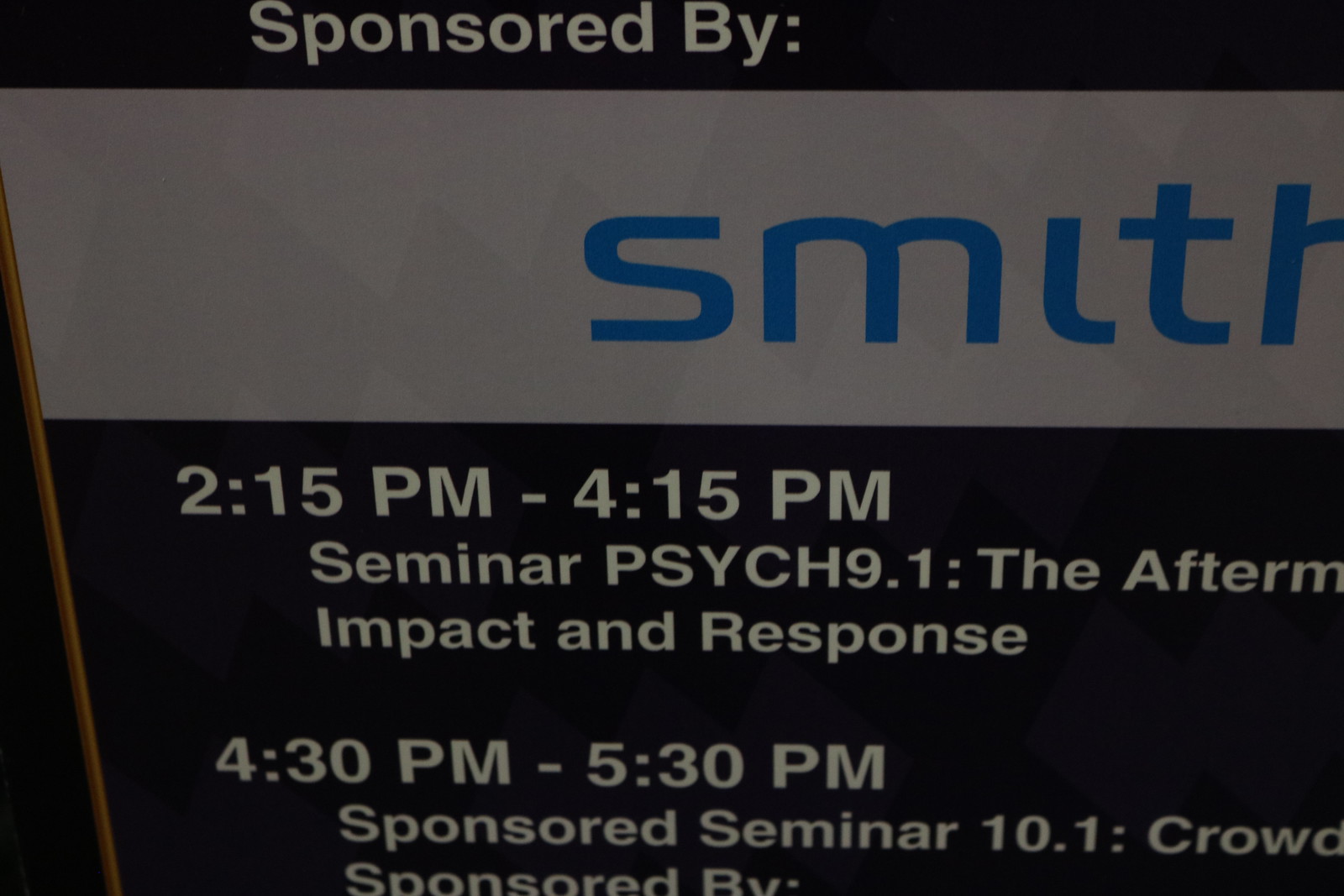The image features a black background with text indicating a schedule for a seminar event. At the very top left, it reads "Sponsored By" in a white sans serif font. Directly below, there is a white banner with "smith" in blue lowercase, sans serif text. Beneath this banner, the background returns to black, displaying the schedule in white sans serif font: "2.15pm to 4.15pm, seminar, psych 9.1, the aftermath, impact and response." Following that, another schedule entry reads: "4.30pm to 5.30pm, sponsored seminar 10.1, crowd." The entire design is framed with a brown border, and the text "Sponsored By" appears again at the bottom, though parts of the image are cropped and not fully visible.